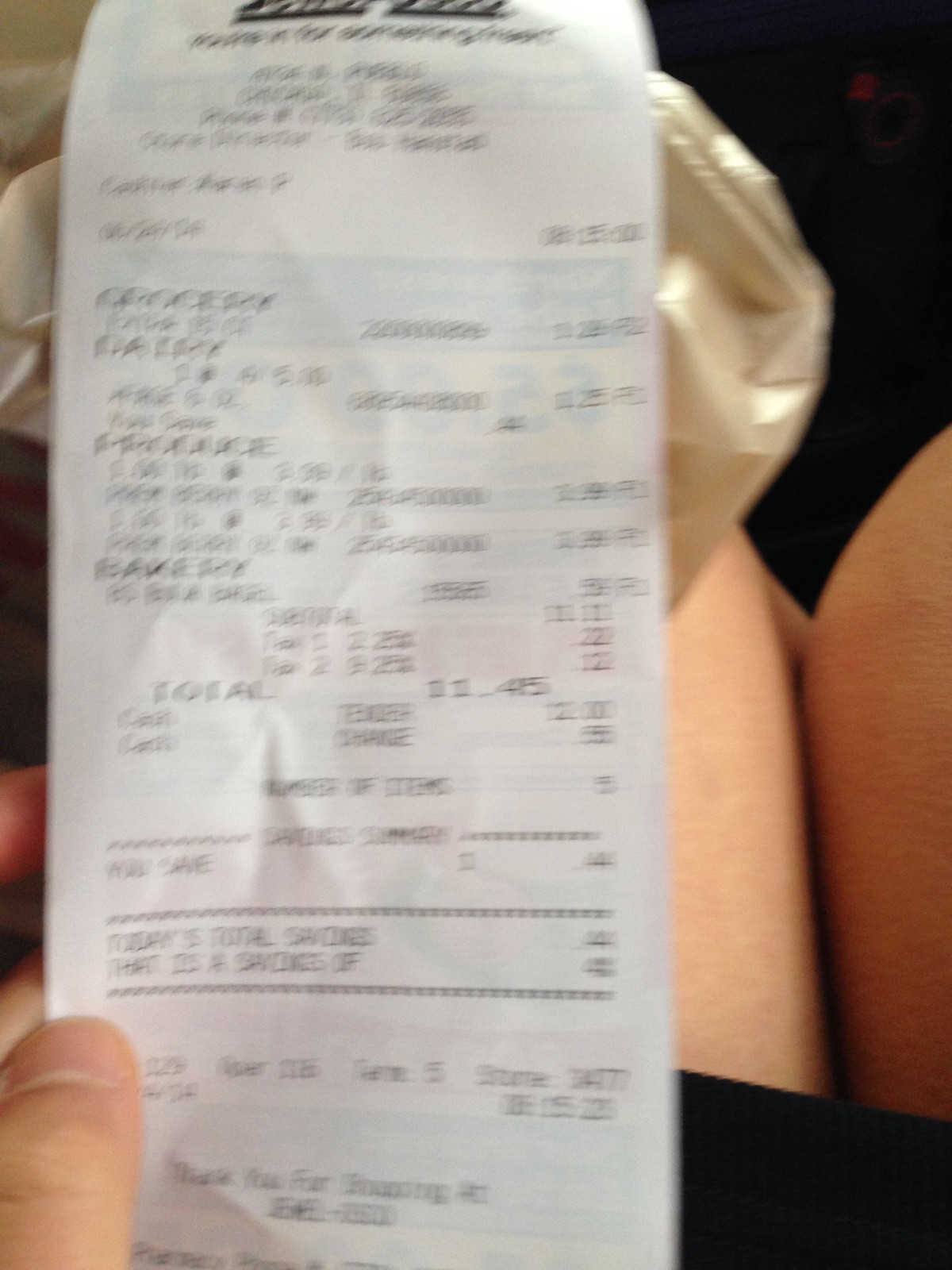The image features a blurred receipt held by a light-skinned hand, with fingers visible in the bottom left corner. The individual holding the receipt is seated, with their light-skinned legs partially visible to the right. They are dressed in a short, dark-colored outfit, possibly a skirt. The top portion of the receipt is cut off, displaying only indistinct dark black print indicating the store name, which is unreadable. Additional store information and details of purchased products, including their prices, are present but also illegible due to the blurriness of the receipt.